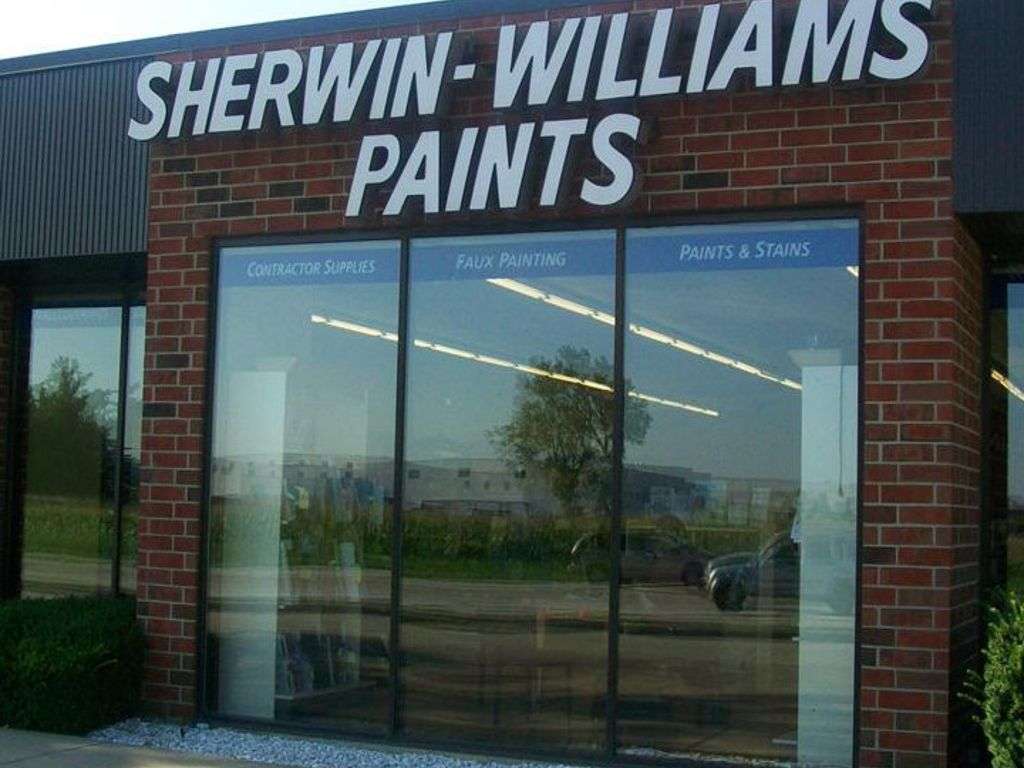This photograph captures the storefront of Sherwin-Williams Paints. The store's name is prominently displayed on a sign that reads "Sherwin-Williams Paints." Below this sign, a large picture window is divided into three sections, each labeled differently: the left section advertises "Contractor Supplies," the middle section promotes "Faux Painting," and the right section highlights "Paints and Stains." The reflection on the window reveals a parking lot in the background, featuring a tree, a building, and two parked cars. Through the glass, you can glimpse the interior where two white bookcases are visible, though their contents are indistinct. The storefront is framed by a brick façade and is flanked by additional windows on either side. In front of the store, a strip of gravel lines the base of the window. The interior is well-lit, with a continuous line of lighting illuminating the space.